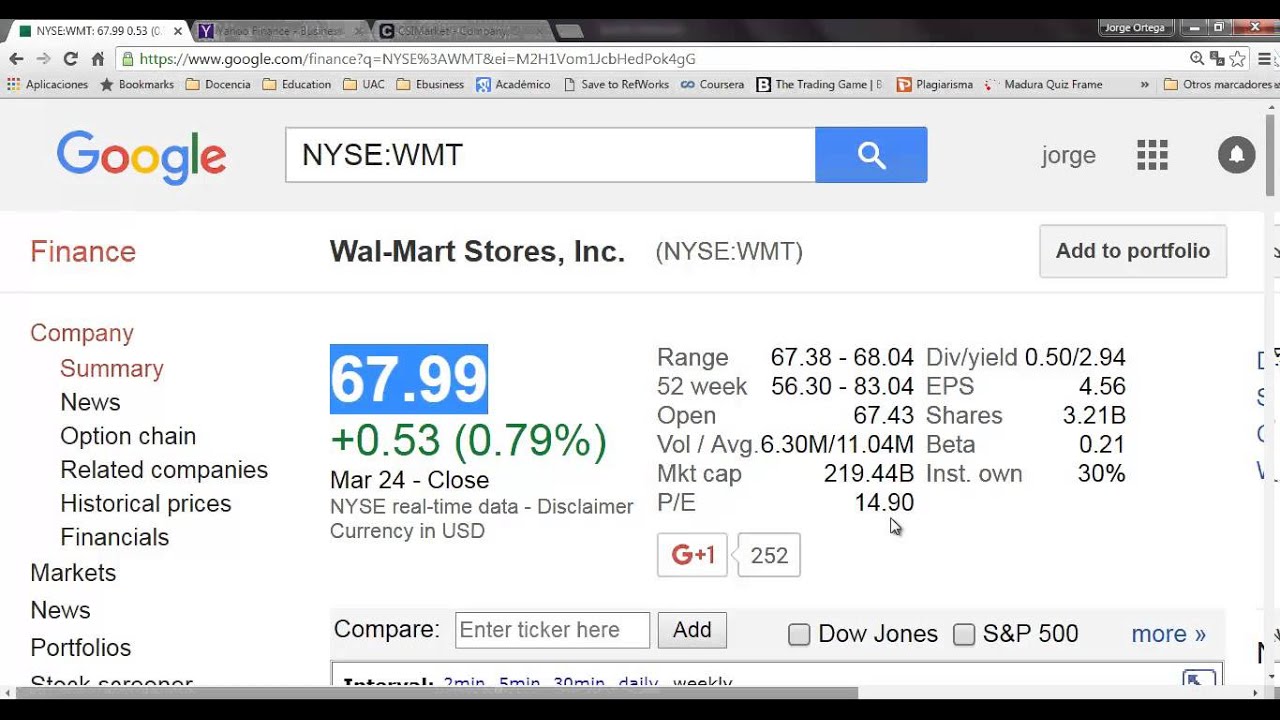The image is a rectangular screenshot of a webpage, approximately one and a half to two times wider than it is tall. At the top of the screenshot, there are three visible browser tabs. The first tab is the active one, displaying what appears to be a Google search. The second tab is a Yahoo page, and the third tab features a logo with a 'C' that isn't clear enough to identify.

The active tab shows the Google logo in the upper left corner, followed by the search bar where the query "NYSE: WMT" is entered. This indicates a search for Walmart's stock information on the New York Stock Exchange. Below the search bar, the main content area features financial data.

In the top left of the main content, there is a red label stating "Finance," followed by the bold black text "Walmart Stores Incorporated (NYSE: WMT)." The stock price is displayed prominently in white text on a blue background. It shows a value of "67.99," with a green indicator below it stating "+0.53 (0.79%)" signifying a rise in stock price. Further down, in black text, it notes "March 27th - Close," specifying the date and the market status.

Overall, the image captures a snapshot of a Google search result page displaying detailed financial information for Walmart's stock as listed on the New York Stock Exchange.